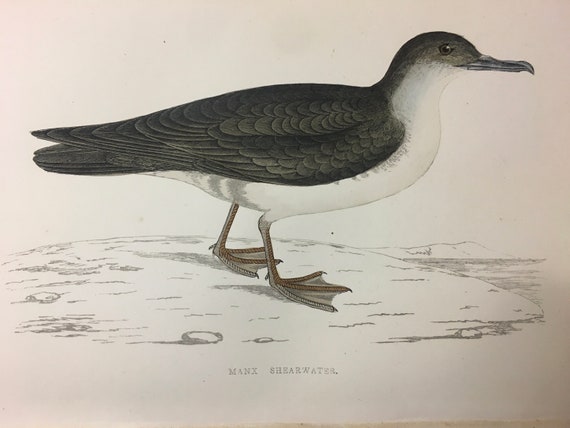This detailed illustration depicts a Manx Shearwater, a type of seabird, rendered in watercolor. The bird is centrally positioned and facing right, possessing a white underbelly, chest, and neck, contrasted by dark gray on its head, back, wings, and tail. The beak is long, thin, and gray with a downward hook at the tip. Its two webbed feet are a distinctive greenish-tan color. The seabird stands on a lightly drawn seashore with marked textures around its feet indicating sand and pebbles, with a hint of water visible on the right. The background is left blank white, ensuring the focus remains on the bird. Below the seabird is a faint, nearly unreadable watermarked name, suggesting the artist's signature.